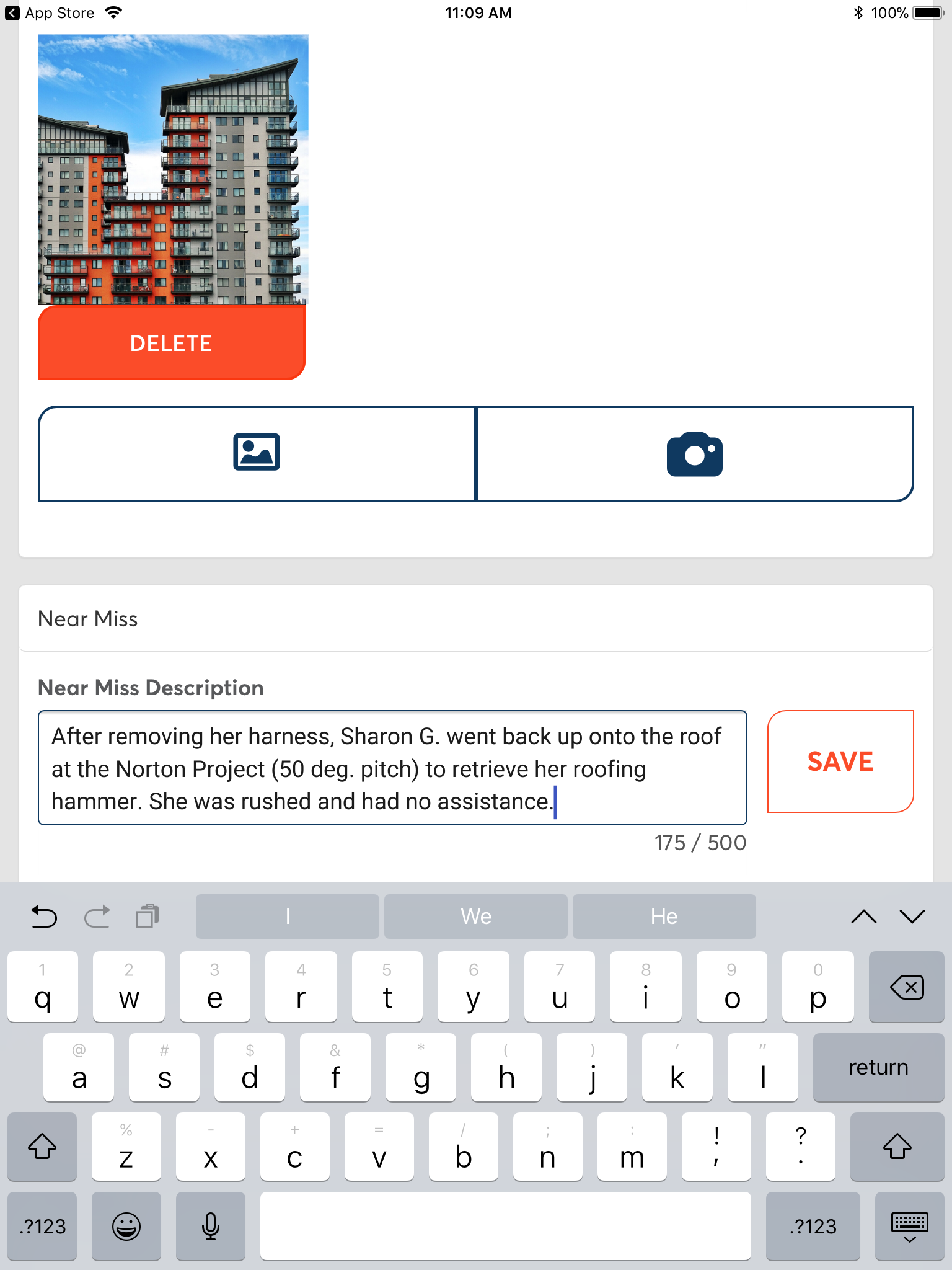The image is a detailed screenshot of a smartphone displaying a page from the App Store, set against a white background. At the very top of the screen, the status bar shows the Wi-Fi symbol, the current time (11:09 AM), the Bluetooth icon, a "100%" battery indicator, and a battery icon.

Centered on the screen beneath the status bar is a photograph featuring four residential skyscrapers with gray and orange exteriors, each adorned with balconies. Notably, two of the buildings have slanted diagonal roofs, adding to their unique architectural character.

Below this photograph, there is a prominent red pill-shaped bar labeled "Delete." Beneath this bar are two navigation tabs: on the left, an icon of a person standing on a mountain, and on the right, a navy blue camera icon. Following these tabs, the text "Near Miss" appears, accompanied by a detailed description. The text recounts a specific incident where Sharon G., after removing her harness, ascended the 50-degree pitched roof of the Norton Project without any assistance to retrieve her roofing hammer.

Further down, the text "175/500" can be seen on the left, with a red "Save" button positioned to its right.

Finally, at the bottom of the screen, there is a condensed keyboard. The keyboard's top row features keys from Q to P and a delete button on the right. The second row contains keys from A to L, with a return button on the right. The third row includes a shift button on the left, keys from Z to M, punctuation marks (exclamation point and question mark), and another shift button on the right. The bottom row hosts several function buttons, including a button leading to additional punctuation options labeled "123," an emoji icon, a microphone button, the space bar, another "123" button, and a button for toggling the keyboard.

Additionally, atop the keyboard are forward and back arrow buttons, along with auto-suggestion options displaying "I," "we," and "he," flanked by up and down arrow buttons.